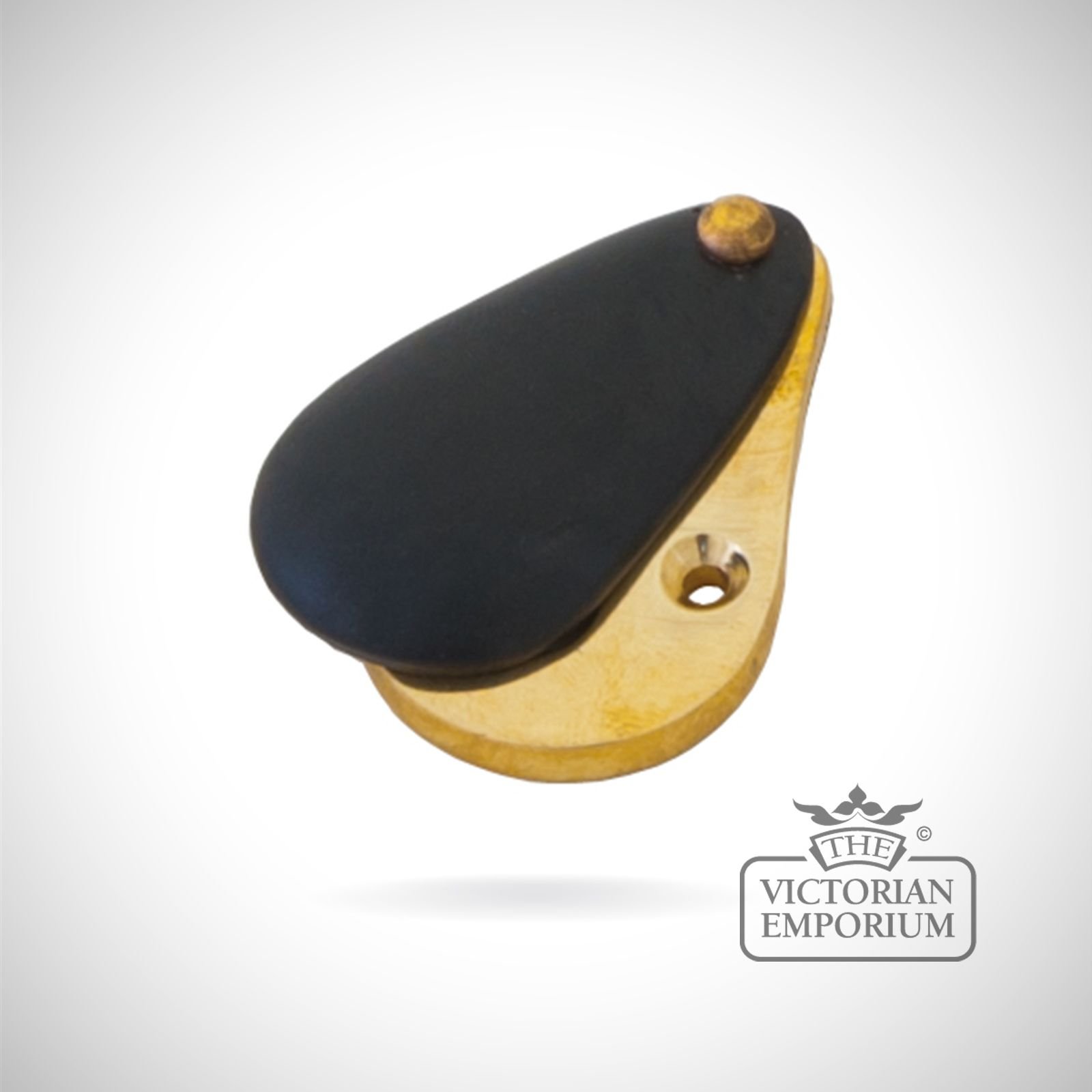The image depicts a Victorian Emporium product, identified by a logo with a crown and a copyright symbol in the bottom right corner. The centerpiece of the image is a pear-shaped device combining wood and black-painted components. The wooden section has a hole in its widest part, while the black top cover resembles a leather slab, similar to a keychain end. The two parts are hinged together at a narrow end by a wooden post. The scene is set against a gray or white background, giving prominence to the craftsmanship and unique design of the object.